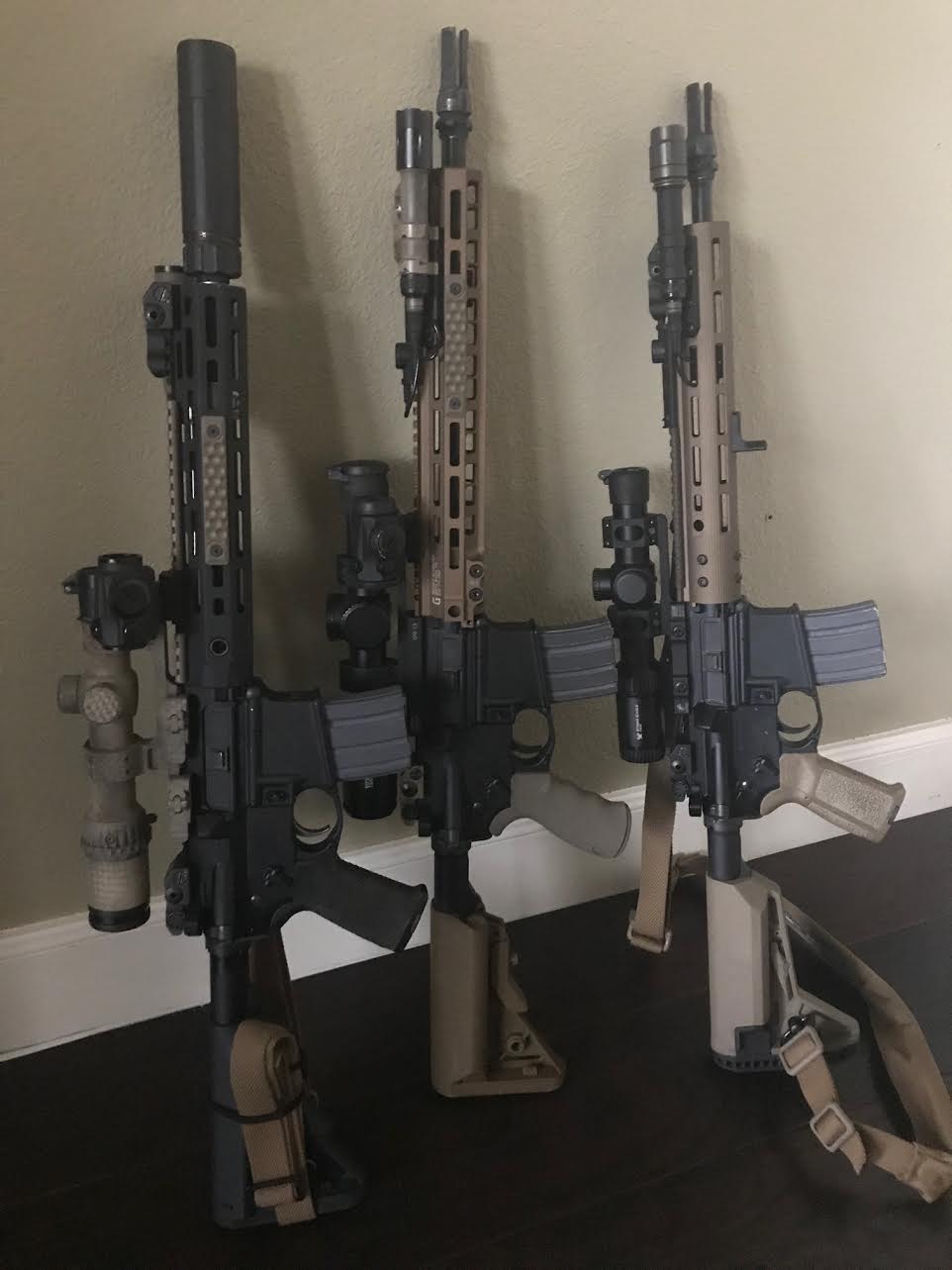This photograph, in portrait orientation, captures three large rifles standing vertically side by side on a dark brown hardwood floor, leaning against a beige wall with a white skirting at the bottom. The rifles, which appear to be semi-automatic firearms, feature various components such as ribbed black magazines for loading bullets and small telescopic scopes for aiming. The rifle on the left is distinctively black with gray and beige details, while the ones in the middle and on the right have a cohesive beige coloring with black accents and handles. Notably, the rifle on the right includes a long beige strap, suggesting it is designed for shoulder carrying. The military-style coloring of the rifles, consisting of shades of gray-green and khaki brown, further adds to their utilitarian appearance.